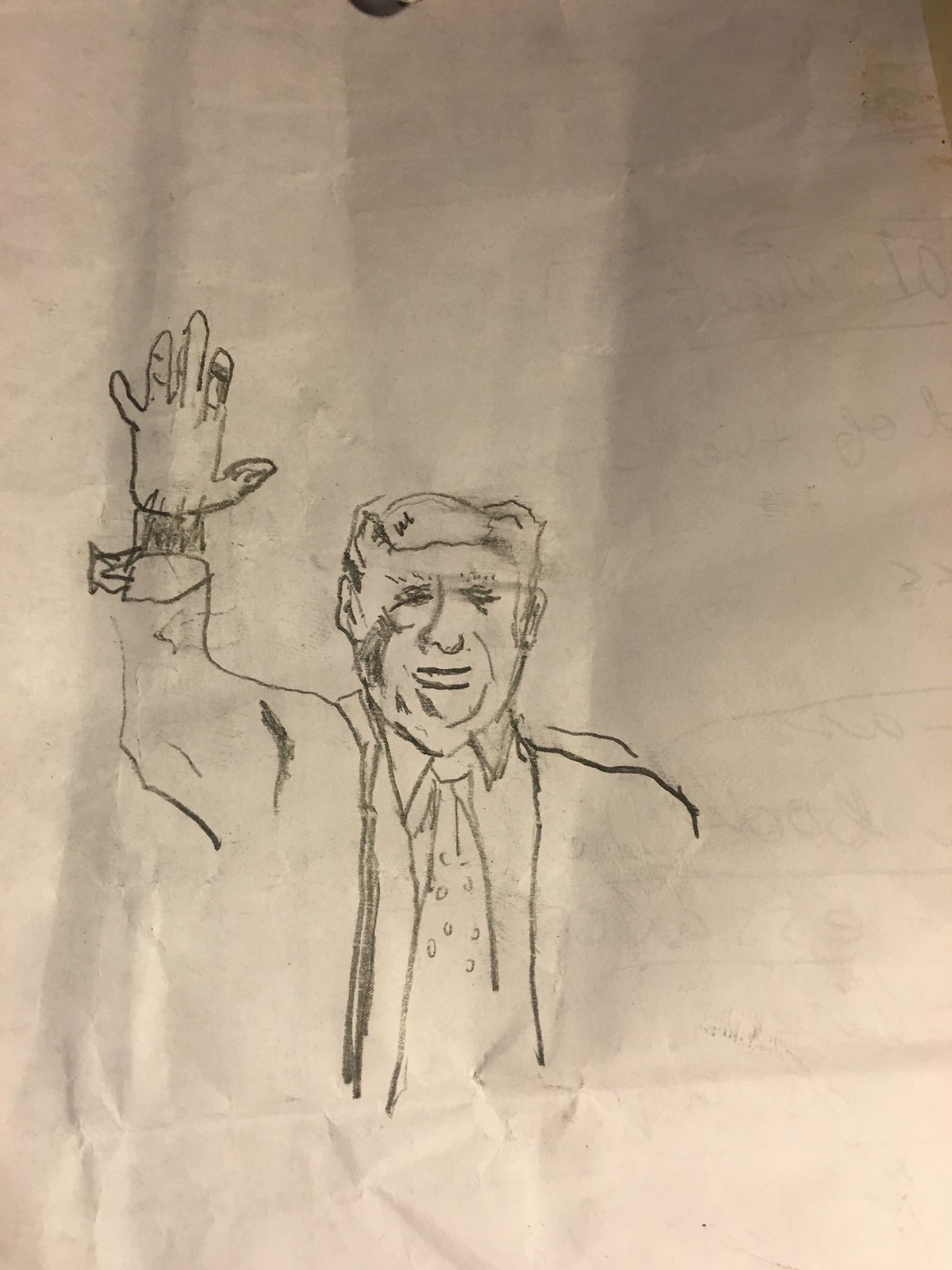This image features a detailed sketch of Donald Trump on a wrinkled white piece of paper in landscape orientation. The paper has faint remnants of mathematical equations, suggesting they were either written on the reverse side or partially erased. The sketch of Trump is positioned at the bottom of the paper, depicting him facing almost directly forward. His right hand is raised in an unusual posture, with the wrist rendered in shaded, squiggly lines, possibly symbolizing something abstract. A shadow falls across the left side of his face, extending over his eyes. Dressed in a suit, Trump sports a tie adorned with spots. His gaze is directed straight ahead, adding to the intriguing nature of the artwork.